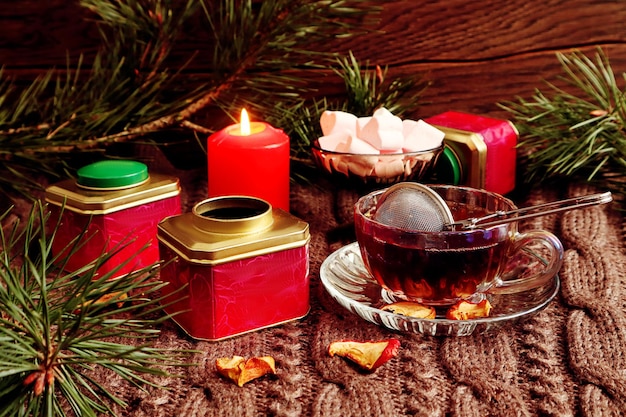The image depicts a detailed Christmas-themed display set on a surface covered with a heavy, brown, knit fabric. Central to the composition is a clear glass teacup filled with a translucent brown liquid, presumed to be tea, with the tea still held in a small mesh strainer attached to a silver handle resting inside the cup. The teacup sits on a saucer surrounded by small pieces of dried apple. 

To the left, there are two metal tins, one open with a gold cap, the other closed with a green cap. A lit red candle sits to the left of the teacup, casting a warm glow. Scattered around the arrangement are branches of pine, invoking a festive, wintry feel. A clear bowl filled with white, heart-shaped marshmallows is visible in the background. The entire setup is backed by a rustic wood grain wall, enhancing the cozy, holiday atmosphere.